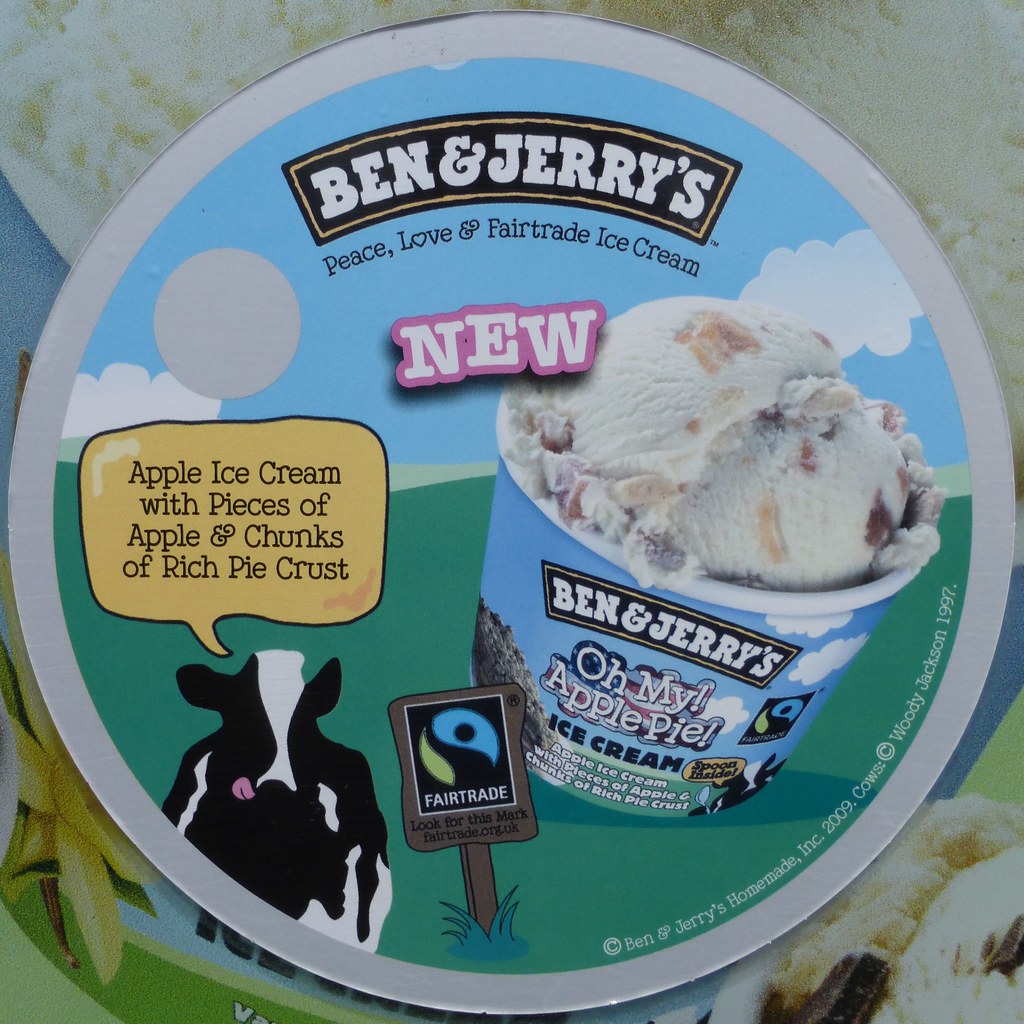The image is an advertisement for Ben & Jerry’s ice cream, specifically their "Oh My! Apple Pie" flavor. The visual layout of the advertisement is designed to look as if you are peering down at the top of an ice cream container. The background appears hazy but depicts a blue sky with two fluffy white clouds. The top of the container prominently displays the Ben & Jerry’s logo, which features white lettering on a black background encircled by a gold band. Below the logo, the slogan "Peace, Love, and Fair Trade Ice Cream" is displayed.

Further down, a pink background prominently highlights the word “NEW,” and beneath it, a green horizon line resembling a field is visible, incorporating shades of light and dark green. To the right of this green horizon, text reads “Apple Ice Cream with pieces of apple and chunks of rich pie crust.” This description is accompanied by an image of the ice cream, showing visible specks of apple and pie crust.

Adding to the details, the advertisement showcases a black and white cow with its tongue playfully sticking out to the right. Beside the cow is a fair trade symbol depicting an arm raised, colored in blue and green with a black silhouette of a human figure. Adjacent to the arm, it states, "Look for this mark, fairtrade.org.uk."

Lastly, wrapping around the top of the label in small print, it indicates "Ben & Jerry’s Homemade Incorporated" with the year 2009 and mentions "Woods Jackson, 1997," whose relevance or exact wording is unclear.